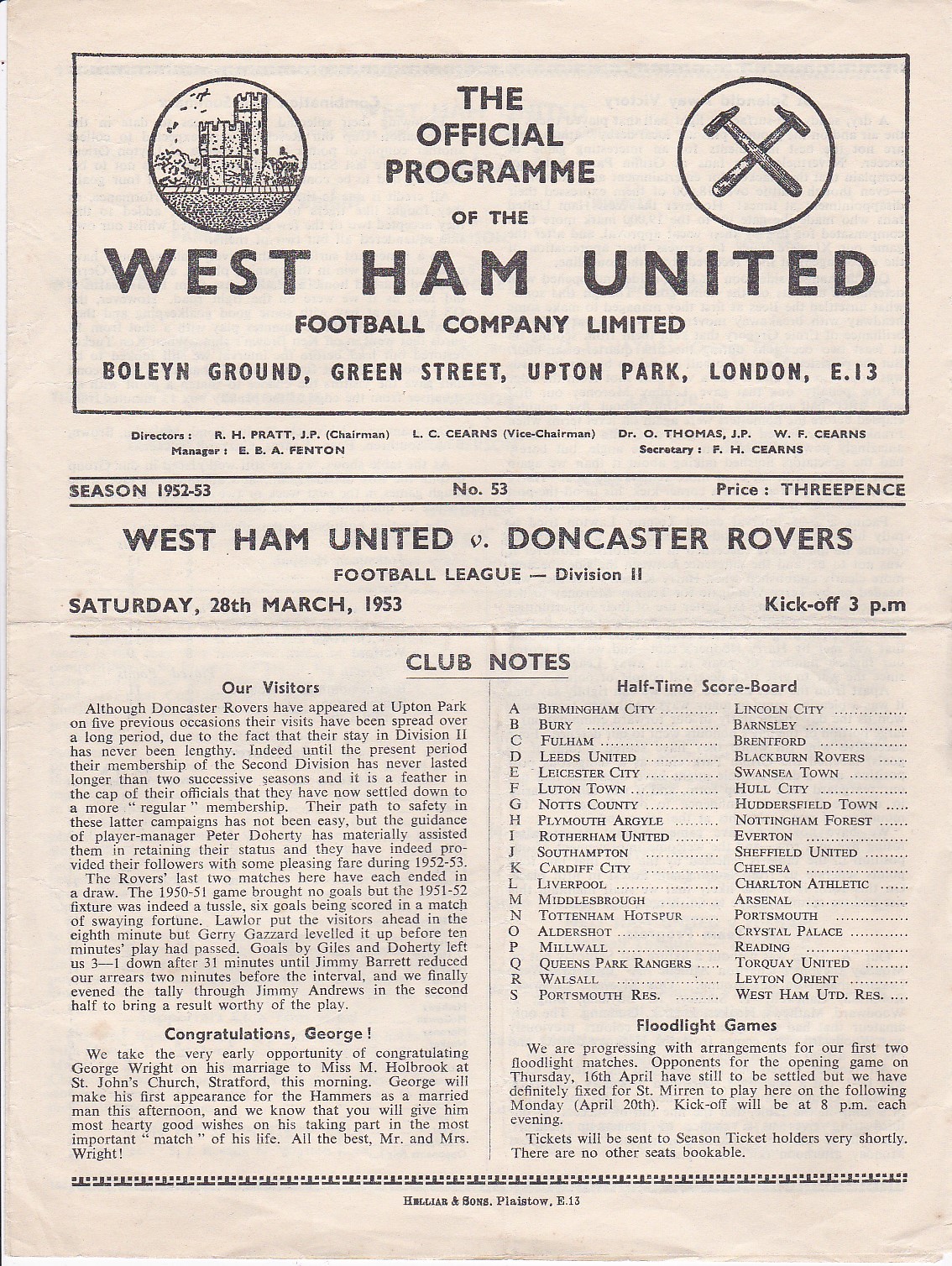This image depicts a beige-colored, possibly cream, official program for the West Ham United Football Club, dating from the 1952-53 season. The program is titled "Official Programme" (with the British spelling), and it's prominently dated Saturday, March 28, 1953, with a kickoff time of 3 p.m. This program covers the match between West Ham United and Doncaster Rovers, held at Boiling Ground, Green Street, Upton Park, London, E13.

At the top of the program, there are two logos: on the left, a small castle, and on the right, two crossed hammers, emblematic of West Ham United. Below this is an array of detailed, small font text, including club notes and information about the visitors. Additionally, there are sections pertaining to "Floodlight Games" and a halftime scoreboard, among other details. The entire text is in a dark gray print, consistent with a typical newspaper cutout from that era.